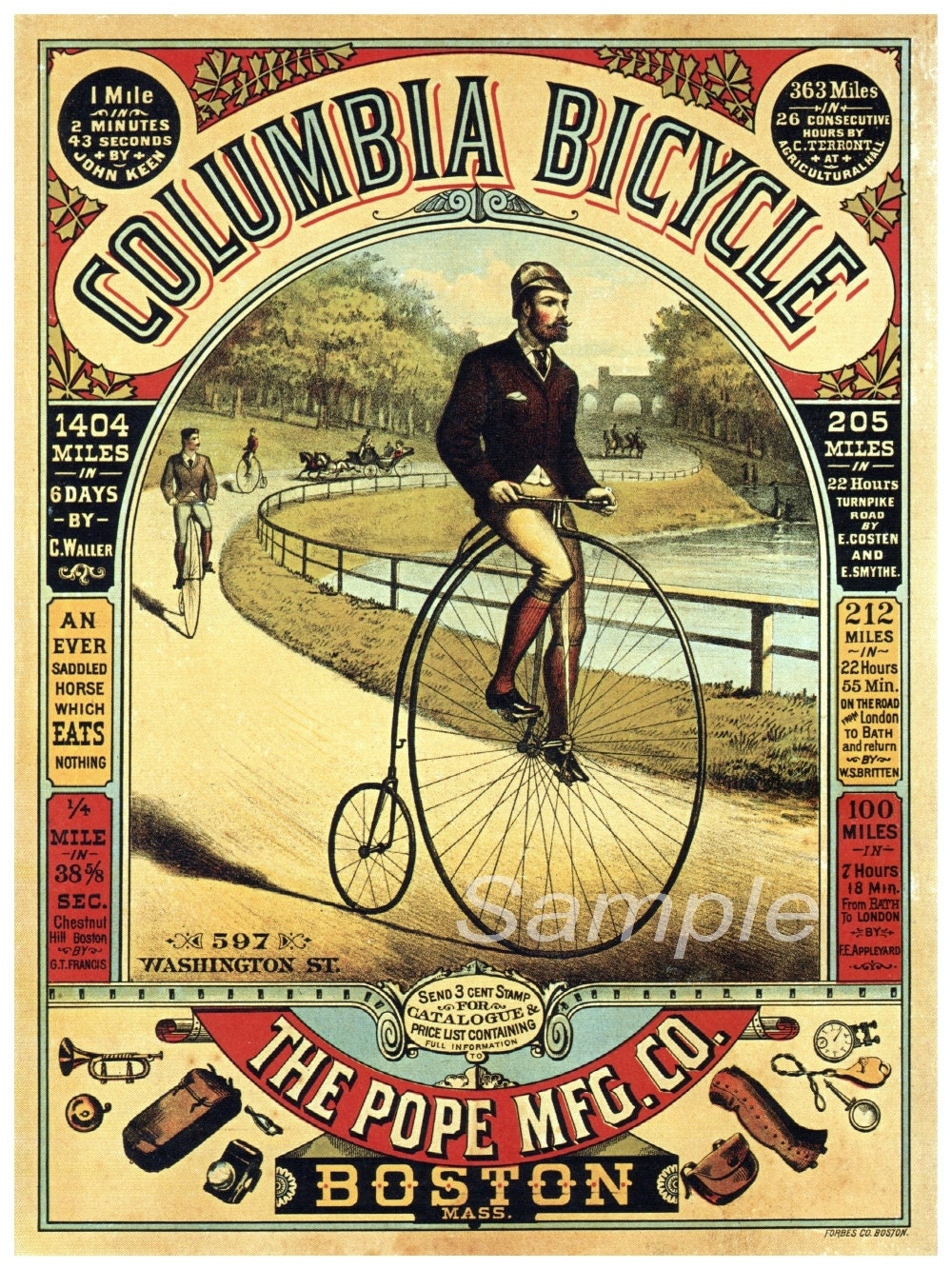This vintage advertisement poster for Columbia Bicycle, produced by the Pope Manufacturing Company of Boston, Massachusetts, features a detailed illustration of a man riding a classic high-wheel "penny-farthing" bicycle. The bicycle has an oversized front wheel, almost taller than the rider himself, and a much smaller rear wheel. The image showcases the rider pedaling along a scenic trail by a river. The poster has a beige background with informational blocks in vivid red, yellow, and black.

Surrounding the central image are numerous records and achievements from various cyclists, emphasizing the bike's performance and durability. Notable mentions include 1,404 miles in six days by C. Waller, 205 miles in 22 hours on Turnpike Road by E. Costin and E. Smith, and a rapid one mile in 2 minutes and 43 seconds by John Keene. Additionally, F.E. Appleyard is credited with covering 100 miles in 2 hours and 18 minutes. These records demonstrate the impressive capabilities of Columbia bicycles and target the adventurous spirit of potential customers.